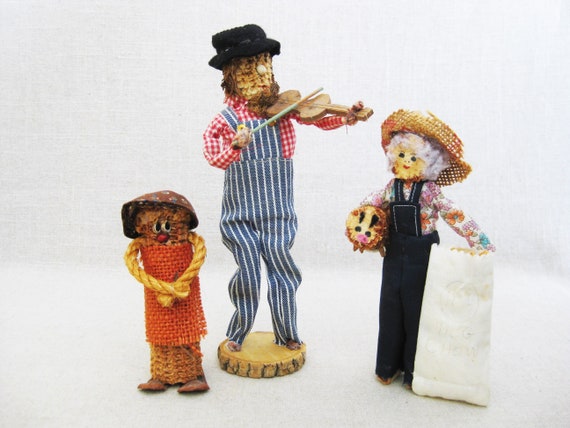This image showcases a set of three handcrafted folk art figurines, meticulously assembled using wood and various other materials. The figurines are set against a white background.

Starting from the left, the first figurine is a creature or stylized old lady, crafted from a cylindrical piece with rope-like arms and adorned with a red top. She holds a small animal, possibly a pig or dog, and has a large sack labeled “Dog Chow.”

In the center stands a man dressed in red and white flannel with blue and white overalls and a black hat. He is portrayed playing a violin, standing on a small wooden stump.

The right-side features another figurine resembling a small girl with hands folded and eyes delicately painted on. She wears a hat and colorful clothes featuring shades of pink, light green, orange, and yellow.

Together, these figures reflect a whimsical and rustic charm, each bringing a unique character to the overall folk art scene.